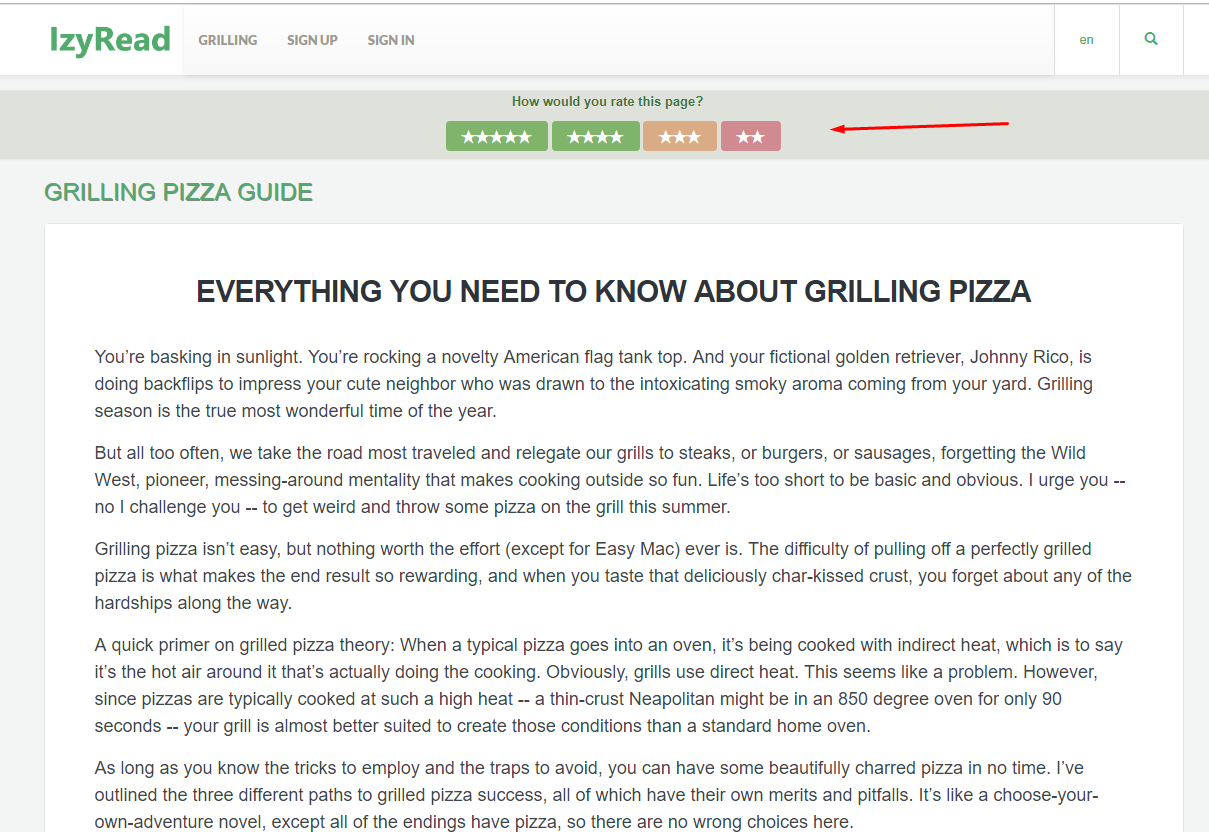Here is a cleaned-up and detailed caption for the described image:

---

The screenshot features a web page titled "LZY Read" with options for users to sign up or sign in. The page prompts users to rate it using a star system, ranging from two to five stars. The primary content is an enticing article titled "Grilling Pizza Guide: Everything You Need to Know About Grilling Pizza."

The narrative sets a vivid scene: Imagine basking in sunlight while wearing a novelty American flag tank top as your fictitious golden retriever, Johnny Rico, performs backflips to impress a cute neighbor, drawn to the tantalizing aroma of smoke wafting from your yard. The article emphasizes that grilling season is the true most wonderful time of the year, encouraging readers to break away from traditional grilling fare like steaks, burgers, or sausages.

It challenges readers to experiment and get creative by grilling pizza, arguing that while it isn't easy, the reward of pulling a perfectly charred pizza off the grill is well worth the effort. The guide dives into grilled pizza theory, explaining that unlike typical pizzas cooked with indirect heat in an oven, grills use direct heat. This might initially seem problematic, but grills can reach the high temperatures necessary for cooking a thin-crust Neapolitan pizza, making them almost better suited for this task than standard home ovens.

The author assures that with the right tricks and the avoidance of common pitfalls, beautifully charred pizzas are just within reach. The guide offers three different methods for grilling pizza, each with its own advantages and challenges, akin to a choose-your-own-adventure novel where every ending involves delicious pizza, ensuring no wrong choices.

The page boasts a clean design with a white background and a light green, greenish-gray border, providing a pleasant and enjoyable reading experience.

---

This detailed caption captures the essence and visual elements of the webpage while inviting readers into its engaging content on grilling pizzas.